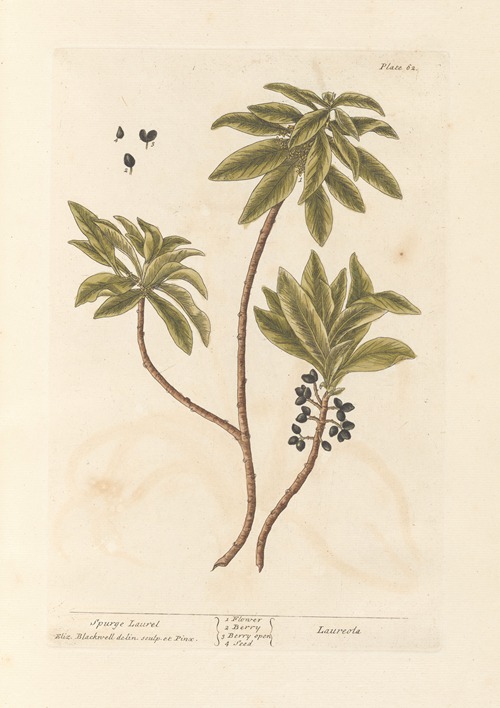The image appears to be a page from an aged botany book with light-colored, yellowed paper. It features a detailed, hand-drawn botanical illustration, likely colored with watercolors. The artwork depicts a plant with two main brown stems. The left stem curves upward toward the center, branching slightly on its left side. The right stem, which also grows upward, has a lower sub-stem and stops just short of touching the upper part of the left stem. Each stem culminates in a cluster of long, narrow leaves. These leaves are layered similarly to a palm tree's, with darker green centers and lighter green edges, and are oval-shaped with pointed tips.

Throughout the illustration, there are small, dark blue to black berries, and possibly some flowers, arranged on the stems. The upper right corner of the page is marked with "plate 6A" in small black letters. Below the illustration, in fine, elegant handwriting, it reads: "Spurge Laurel," followed by the name "Eli Blackwell," and a possible sequence indicating different parts of the plant, including "1 flower, 2 berry, 3 berry open, 4 seed."